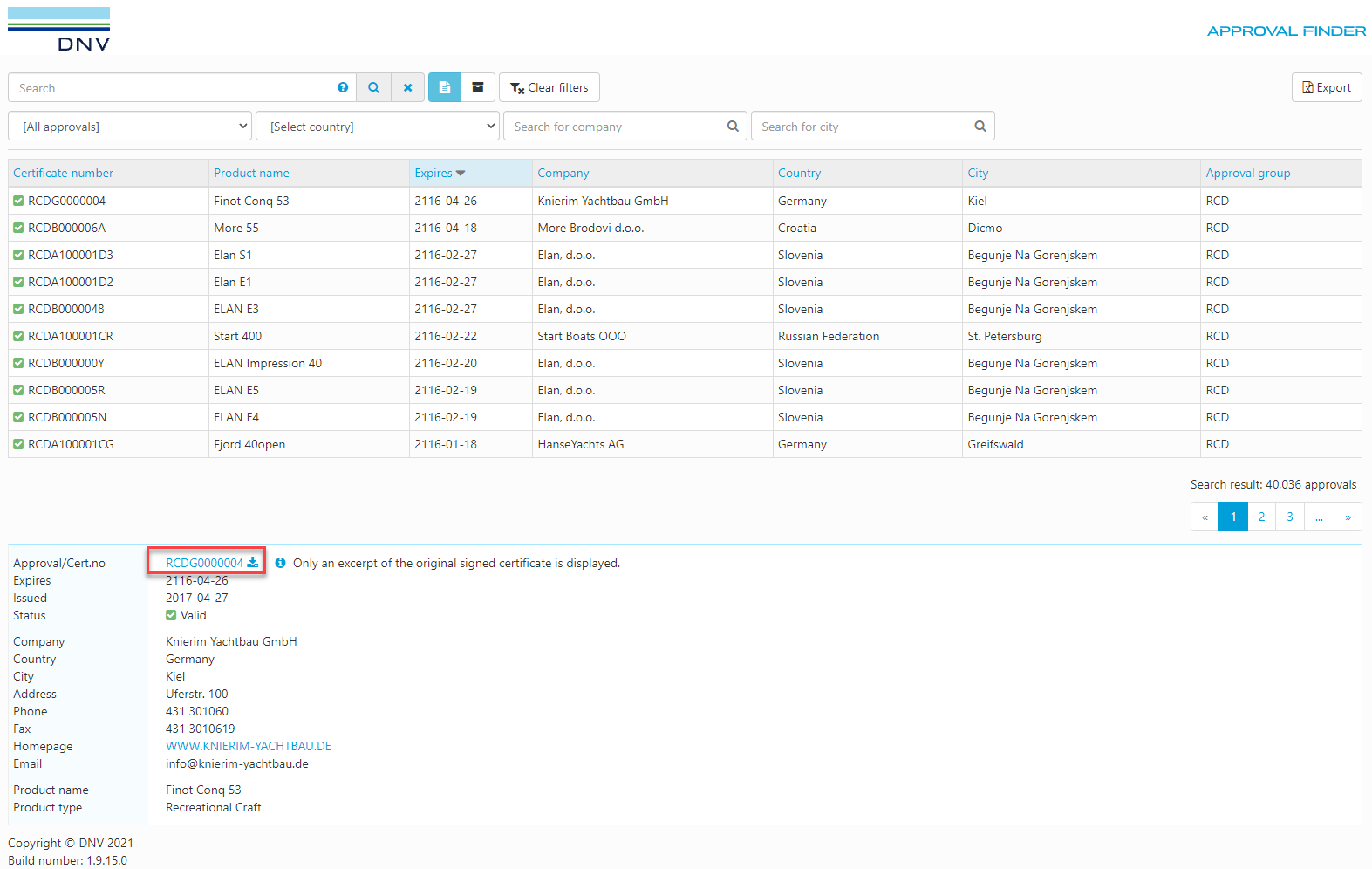In the image, at the top left corner, the logo 'DNV' is prominently displayed. The layout includes several columns and rows, each serving a specific purpose. The first column lists approval statuses, the second allows for country selection, and the third deals with forwarding options. Within the table, columns are labeled as follows: the first column displays certificate numbers, the second shows product names, the third indicates the expiry dates, the fourth lists companies, the fifth details the country of origin, the sixth marks the cities, and the seventh denotes the approval group.

Above the table, the header features options for 'All Approvals,' 'Select Country,' 'Search for Company,' and 'Search for City.' In the top right corner, there is a search box titled 'Approval Finder.' At the bottom left of the image, the text 'ROCDG0000004' is highlighted in red, drawing attention.